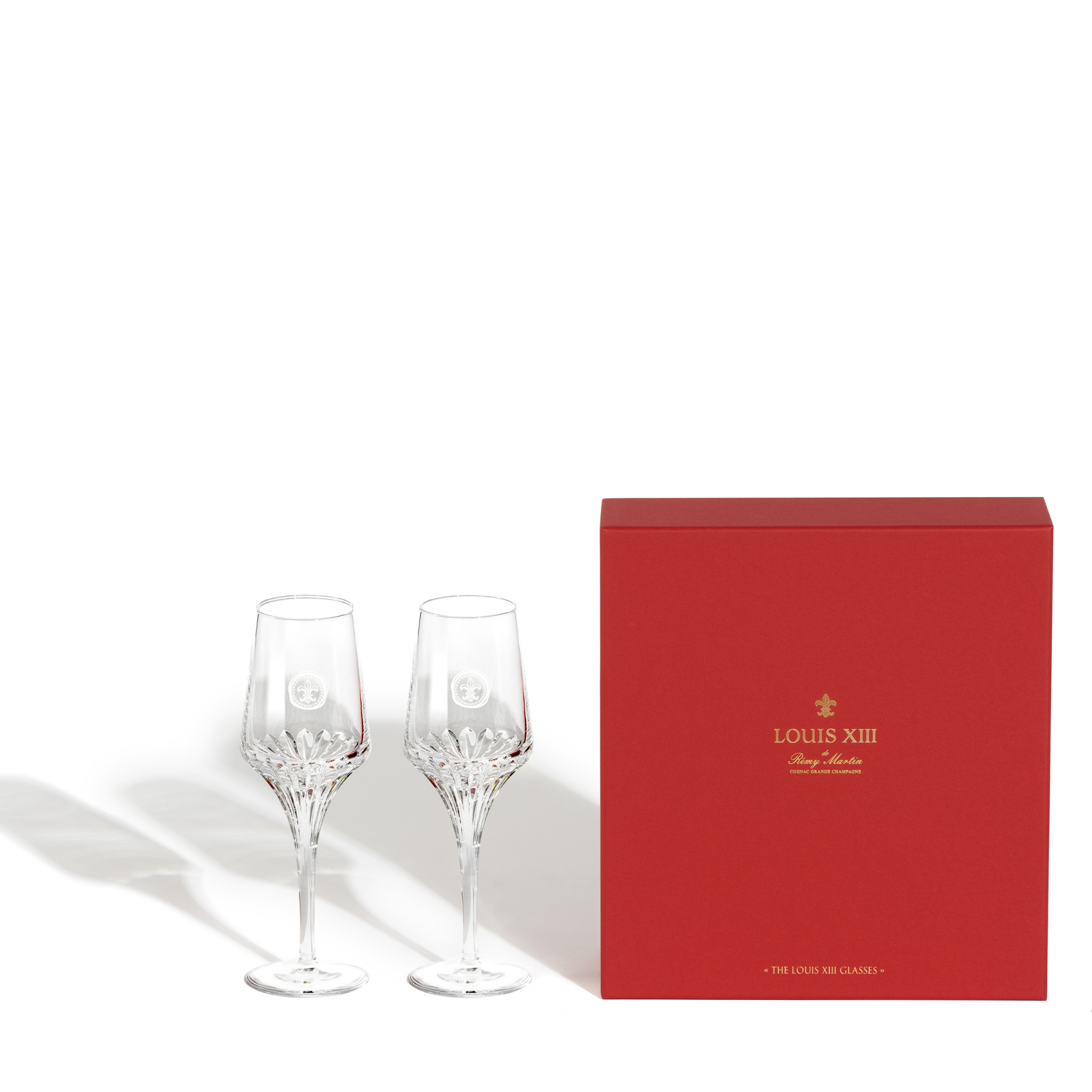The image showcases an elegant set of Louis XIII wine glasses. To the left, there are two long-stemmed crystal wine glasses, each adorned with intricate, jagged designs at the base of the stem and a circular etching resembling the emblem found on the box. The glasses cast their shadows against a pristine white background. To the right, a striking, bright red square box stands prominently, featuring the text "Louis XIII" in gold lettering at the center, accompanied by a decorative gold filigree above it. The bottom of the box has additional small lettering that is difficult to make out. This box is likely the packaging for the sophisticated wine glasses. Both the glasses and the box add a touch of luxury to the scene.